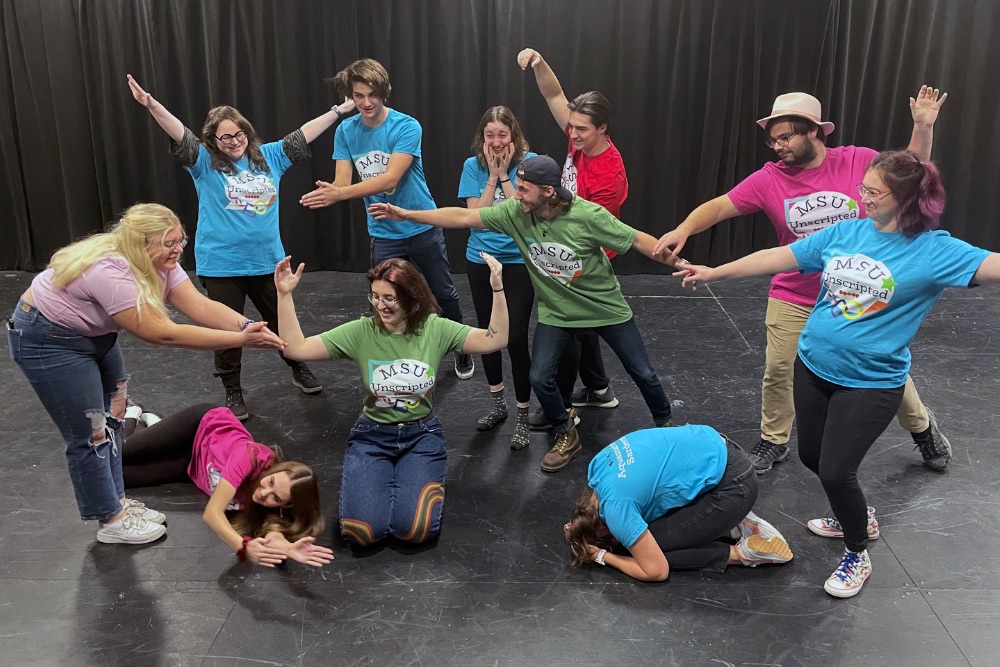This full-color indoor photograph captures a lively scene from a college theater class or an unscripted improv group at Michigan State University (MSU). The artificial lighting brightly illuminates the square image, which features a gray, scuffed-up stage floor and a backdrop of black curtains. The diverse group of young, Caucasian men and women is dressed in a variety of colorful crew-neck T-shirts emblazoned with "MSU Unscripted," in hues including blue, green, red, pink, orange, and gray. 

Positioned at the center, three individuals are on the floor; one woman is on her knees with her hands raised, while two others, a man and a woman, are bowing down beside her, all with infectious smiles and laughter, suggesting a fun and engaging routine. Surrounding them, other members of the group stand in a semicircle, some with arms outstretched and expressive faces, enhancing the dynamic and spontaneous atmosphere of the scene. The men in the group include a few wearing hats, adding to their casual, yet spirited ensemble. This snapshot vividly portrays the energy and camaraderie of an MSU improv dance comedy performance.